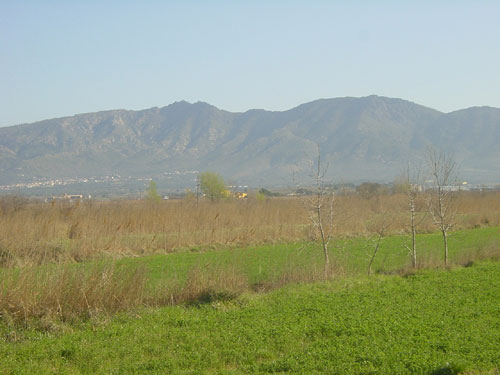The photograph depicts a serene open field with a mixture of lush green grass and rows of taller brownish grass or weeds. Scattered across this landscape are four small trees, all bare of leaves, likely due to the winter season. The foliage is green but not perfectly manicured, and there are distinct diagonal strips alternating between green and brown vegetation. In the background, a slightly taller bush or shrub stands out before the terrain transitions into rolling foothills. Beyond these foothills, a small mountain range spans the horizon beneath a hazy blue sky. Though the day appears clear, the atmosphere carries a slight fog, rendering the distant peaks somewhat opaque. At the base of the mountain on the left side, one can discern the faint outline of a village or town, with buildings and possibly cars, adding a human element to the otherwise untouched natural landscape.